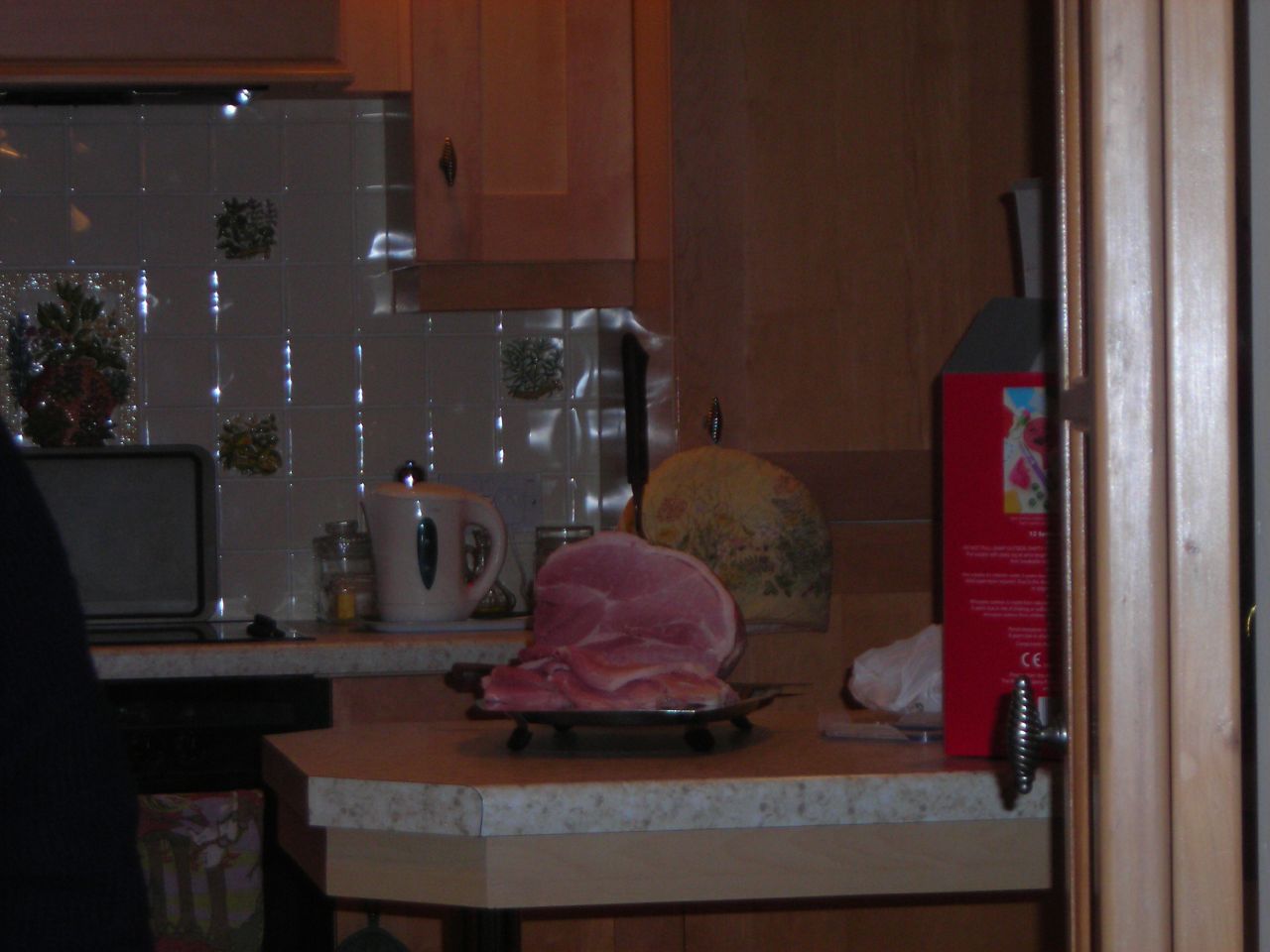This photograph captures a cozy, old-style kitchen with light tan cabinets and a white tiled backsplash. On a white-patterned countertop sits a platter with a partially sliced ham, with several slices placed neatly in front of it. The scene is framed by a dark wooden doorframe on the right. In the background, besides the backsplash, a white kettle and stovetop can be spotted. The overall tone of the image is warm and welcoming, characterized by a blend of brown and white hues.